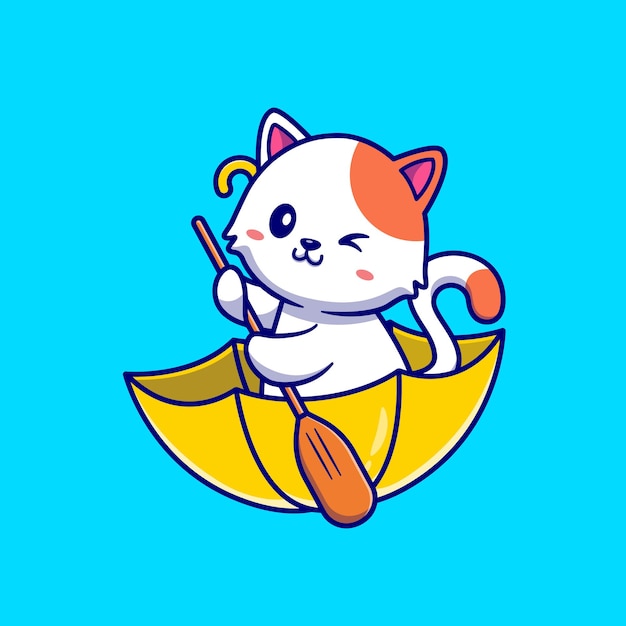In this detailed color image, we see a charming cartoon cat engaging in an imaginative adventure. The cat is predominantly white with distinctive orange patches on its upper left ear, forehead, and the tip of its tail, which curves out from the rear on the right side. The cat's facial expression includes one open eye on its left and a closed eye on its right, giving the appearance of a playful wink. The cartoon feline’s nose is black, and its mouth curls upwards into a smile. Additionally, it features two pointy ears with pink insides, one of which is orange on the outside while the other is white. The cat also has blush-like oval shapes on its cheeks in a reddish-orange hue.

This adventurous cat is seated in an inverted yellow umbrella, with the cane handle curved and arching up on the left side, seemingly transforming it into a makeshift boat. The yellow umbrella itself is outlined in blue, and the entire scene is set against a solid sky blue or turquoise background. The cat is depicted with a brown paddle in its paws, with its left paw positioned lower than the right, suggesting the cat is actively rowing its whimsical vessel. The cartoon is outlined in blue, completing the playful and engaging atmosphere of the illustration.